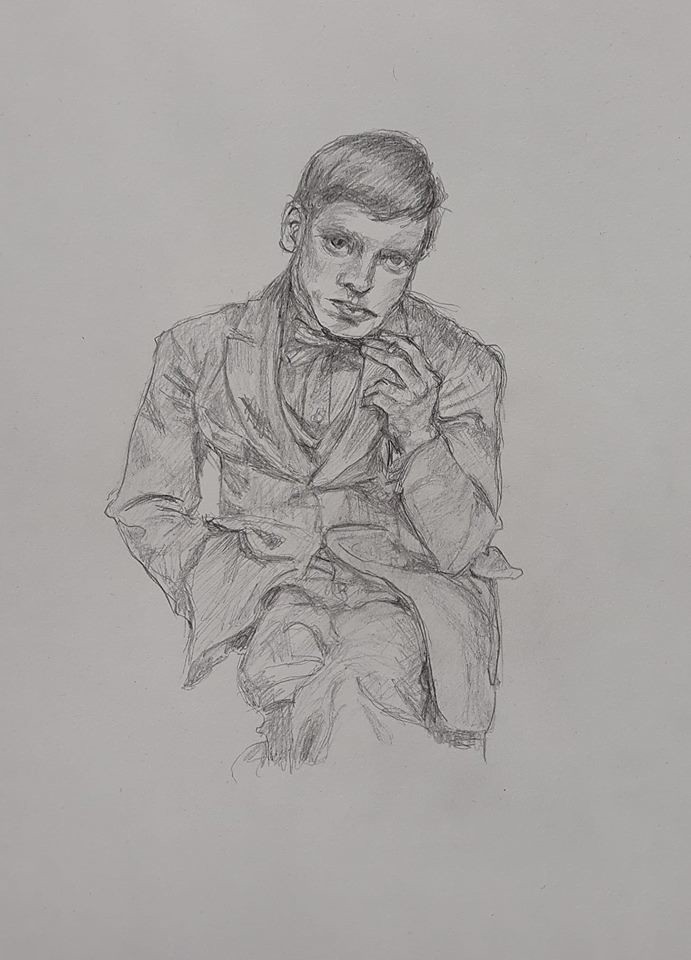The image is a pencil drawing set against a white background. It depicts a man who appears to be an esteemed scientist or astronomer, potentially resembling the late Stephen Hawking. The subject has short hair, neatly combed to the side, though the pencil medium precludes determining its color. He is clad in a suit, with a bowtie adding a touch of formality. His left hand, which appears on the right side of the image, is holding an object between the middle and index fingers—possibly a pen or cigarette. Meanwhile, his other hand is obscured, tucked into what might be a suit or pants pocket. The drawing captures a moment of poised contemplation or readiness, typical of a figure of intellectual rigor.